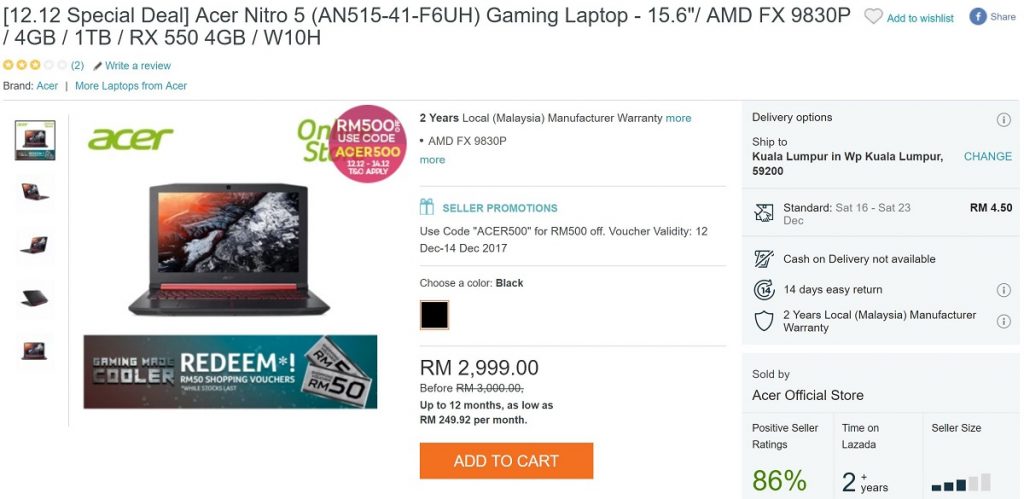A screenshot of a website's purchasing page features a sleek black gaming laptop with a distinctive red stripe. The focal image shows the laptop open, displaying an abstract design with hues of red, white, and black on the screen. Additional smaller images on the left provide various angles of the laptop. A banner beneath these images states "Gaming Made Cooler," promoting a deal for RM 50 shopping vouchers and includes two small voucher icons labeled RM 50.

At the top of the page, a bright pink circle highlights a special offer: "RM 50 or RM 500," with the code "Acer 500." Above this is further laptop information reiterated in the banner. Users can add the item to their wish list by clicking a heart icon, while a blue circle with an "F" provides a link to share the page on Facebook. An orange "Add to Cart" button with white lettering is prominently placed, and next to it, a blue "Seller Promotions" button featuring a present icon can be found. The laptop is priced at $2,999.